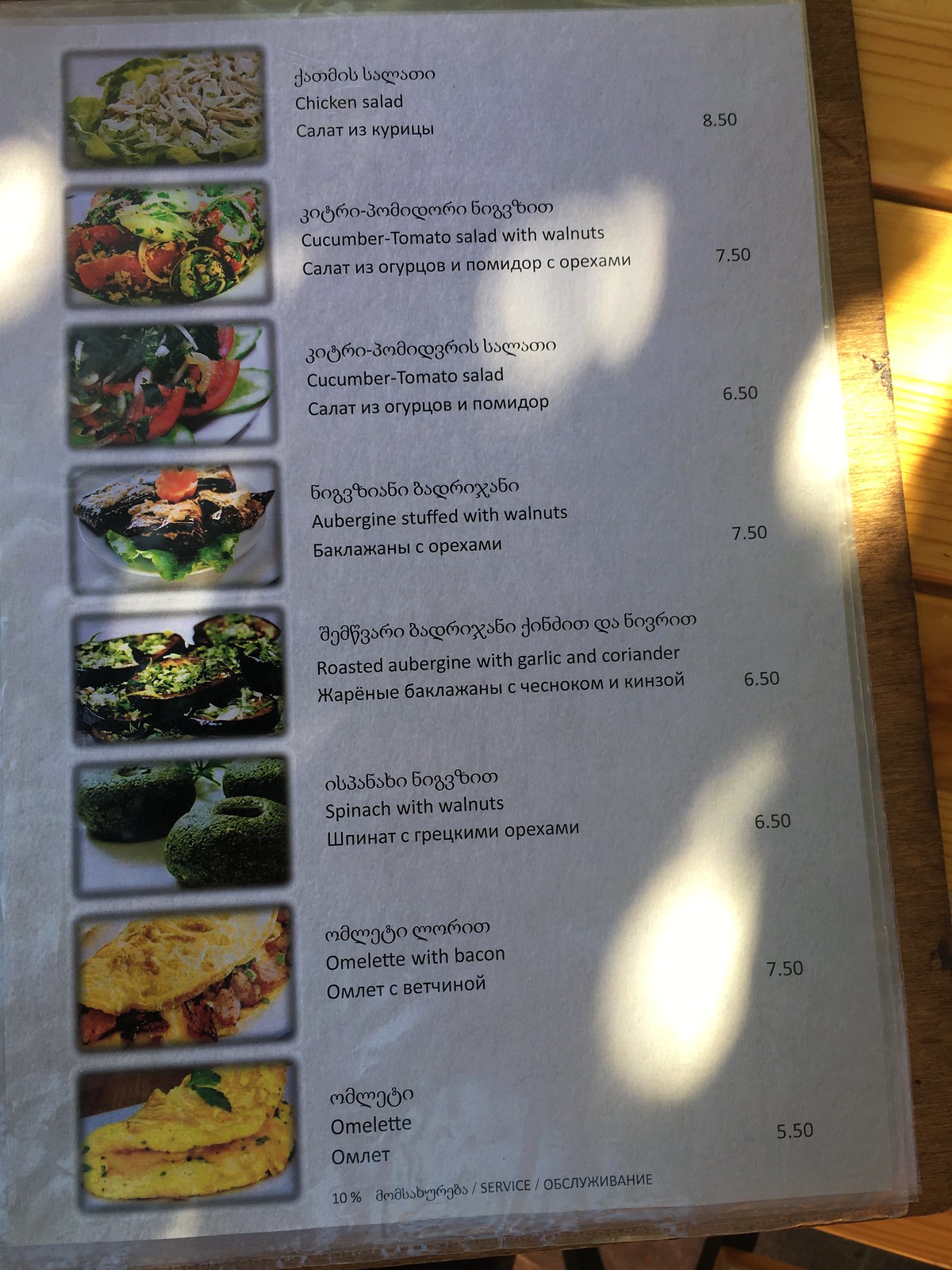The image depicts a segment of a menu placed on a light brown wooden table or bench. The menu itself is white and features food items listed in three different languages: English in the middle with another language above and below the English text.

The items listed in the menu include:

1. **Chicken Salad** - Priced at $8.50, it is described with an accompanying image showing the salad served on a bed of lettuce with possibly some avocado.

2. **Cucumber Tomato Salad with Walnuts** - Priced at $7.50, it features a picture with tomatoes, cucumbers, onions, and nuts.

3. **Cucumber Tomato Salad** - Priced at $6.50, the picture shows cucumbers, tomatoes, onions, and greens.

4. **Aubergine Stuffed with Walnuts** - Priced at $7.50, possibly described with a picture of brown mushrooms stuffed with walnuts, served on a piece of lettuce on a white plate.

5. **Roasted Aubergine with Garlic and Coriander** - Priced at $6.50, depicted as mushroom caps filled with green and white ingredients.

6. **Spinach with Walnuts** - Priced at $6.50, described with an image showing dark green spinach shaped like doughnuts.

7. **Omelet with Bacon** - Priced at $7.50, shown as a yellow egg omelet stuffed with bacon and possibly other ingredients like onions.

8. **Omelet** - Priced at $6.50, depicted as a regular egg omelet with a small leaf on top, possibly mint, and stuffed with what might be cheese.

At the bottom of the menu, there's a note mentioning a 10% service charge. The back of the menu appears to be dark brown.